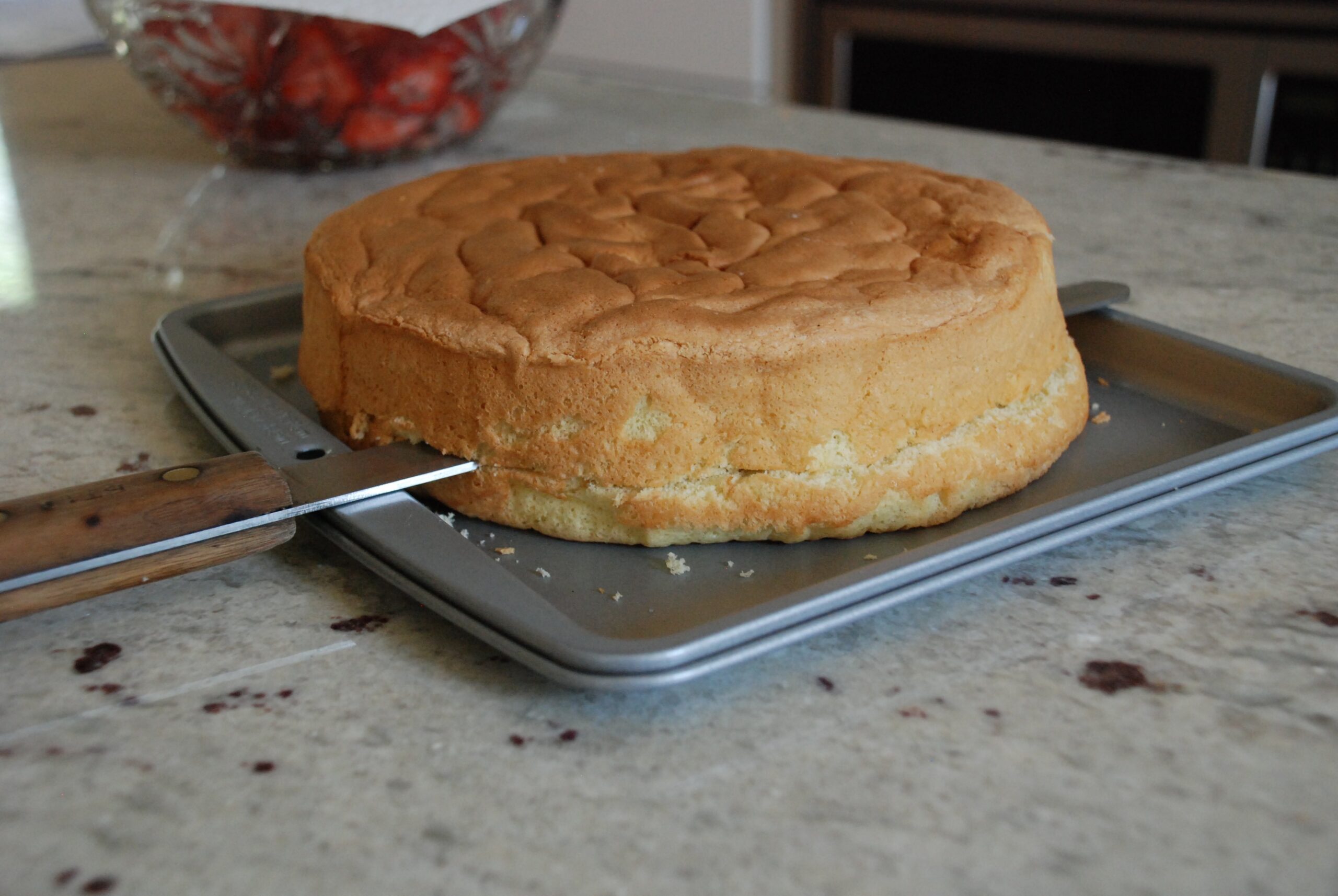In the foreground, a golden brown cake, approximately six inches in diameter, sits on a silver baking sheet atop a marble countertop with red flecks. A long knife is cutting horizontally through the cake, suggesting it has just been taken out of the oven. To the right of the cake, there is a glass dish covered with a napkin, containing a mix of strawberries and blueberries. Additionally, a small bowl filled with similar fruit sits nearby. In the slightly blurred background, the shadows of two black chairs can be seen against the marble counter, adding depth to the kitchen setting.